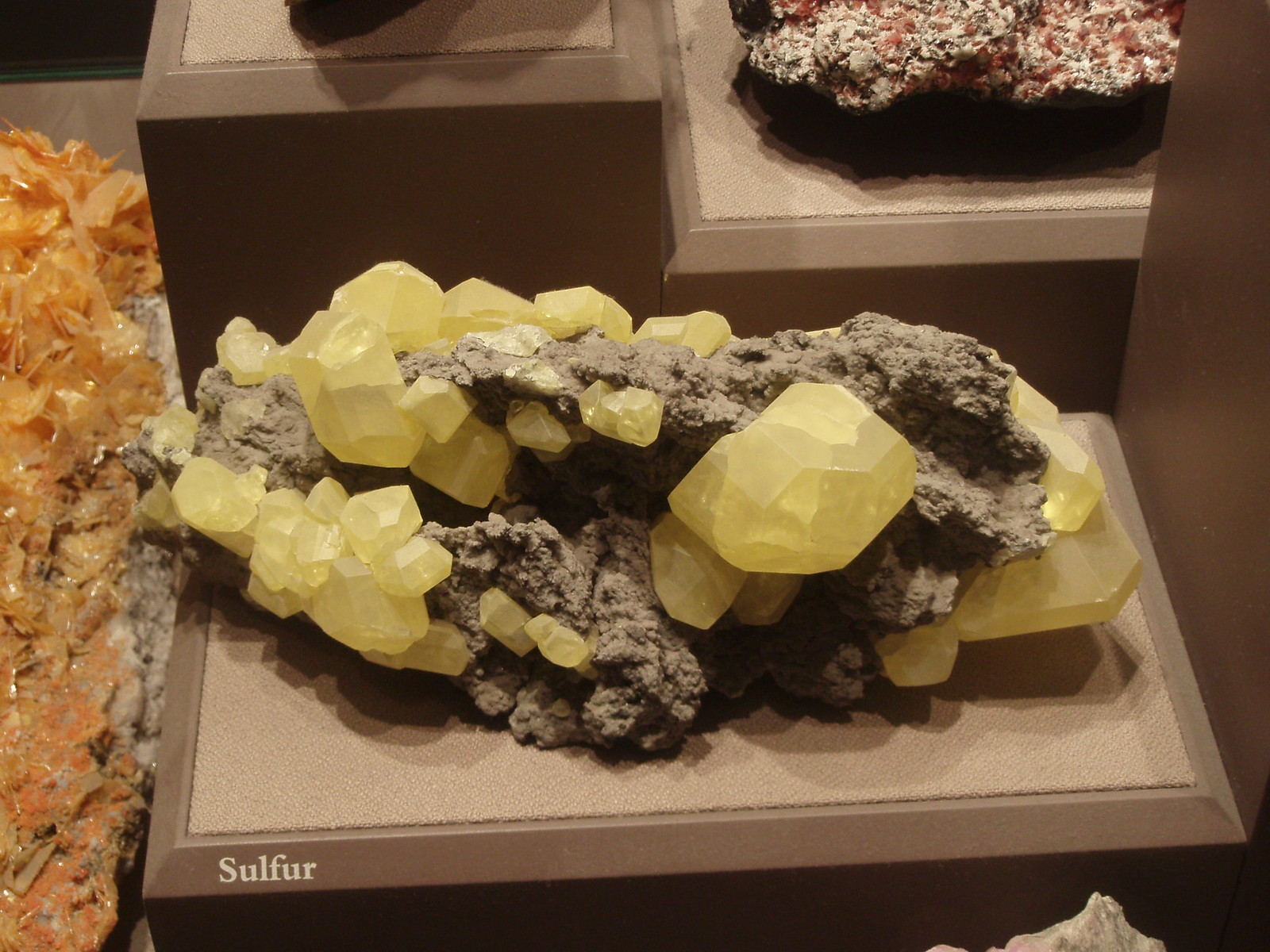This image depicts a museum display featuring a large, irregularly shaped gray rock encrusted with vibrant yellow sulfur crystals. The rock, along with the sulfur crystals of varying sizes, rests on a textured light brown platform. The base of this display has the word "sulfur" printed in white letters on the bottom left. To the left of the main sulfur display, there is an additional crystal, which is a combination of orange and peach hues. The background of the image reveals multiple other platforms, unlabelled, showcasing different types of materials, including a rock that is red, black, and white in color. This structured and educational setup suggests it is designed for informative purposes, possibly within a museum.